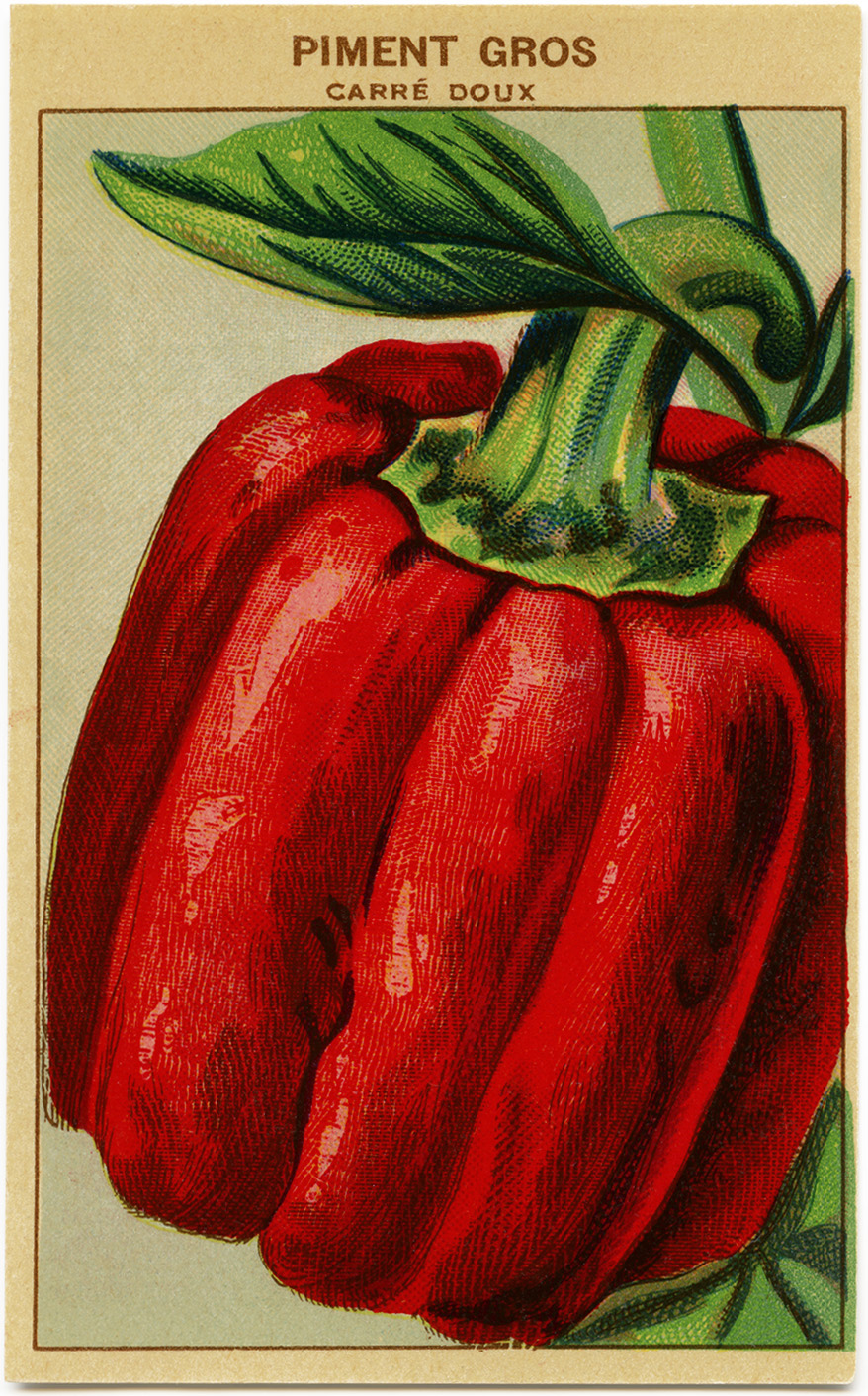This depiction shows a highly detailed and dynamic illustration of a red bell pepper. The painting features vibrant colors, with a very red bell pepper highlighted with pink shades and outlined in black to emphasize its contours and ridges. The bell pepper is attached to its green stem, from which extends a dramatic and dynamic green leaf, featuring black contours and yellow highlights. The overall texture of the image suggests a combination of colored pencil and ink, with a potential for it being a print due to smaller dot patterns.

The artwork is framed with a beige border and contains brown lettering at the top, spelling out "Piment Gros Caridou" in French. This might indicate the name of the pepper variety or could suggest a seed packet design. The wording is split with "P-I-M-E-N-T-G-R-O-S" on one line and "C-A-R-R-E-/D-O-U-X" underneath, highlighting the detailed and ornate nature of the illustration. The background of the illustration is done in a color akin to cardboard, lending a vintage or rustic feel to the presentation.